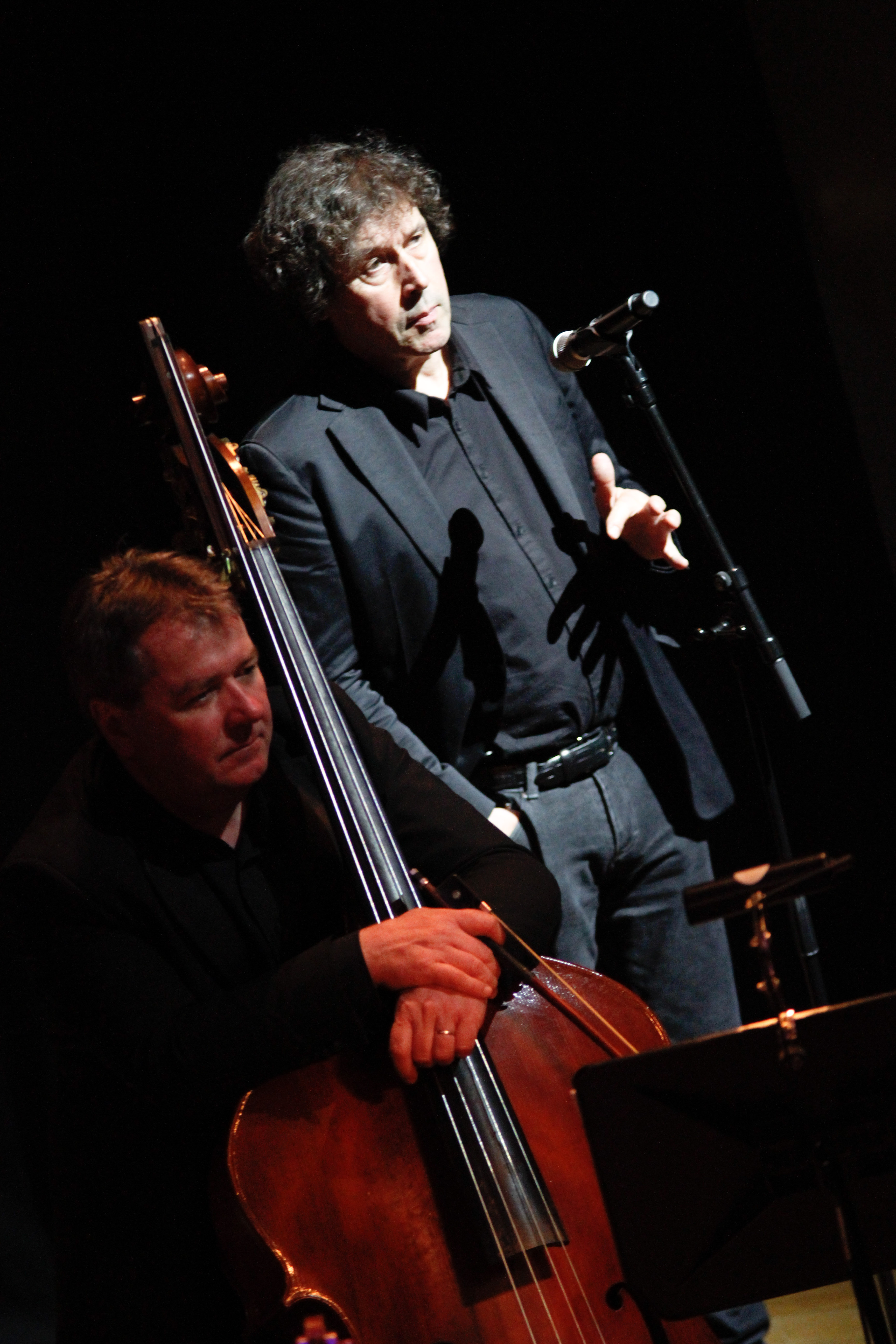In a tall, rectangular photograph with a very dark background, two men are captured mid-performance, appearing slightly tilted from the bottom right corner to the top left. The taller man stands to the right, clad in a dark button-up shirt, a sport jacket, blue jeans, and a shiny black belt. His presence is accentuated by his curly brown hair and a tall microphone positioned in front of him as he listens attentively. Beside him, seated in the bottom left corner, the other musician, with reddish hair barely visible under the shadows, dons a dark long-sleeve shirt. His hands delicately wrap around a large cello, its dark shiny brown body extending far above his head with the handle reaching towards the top left corner. The cello player appears to be concentrating intensely, possibly on a sheet of music before him, as both musicians share a moment of attentive stillness in the midst of their performance.